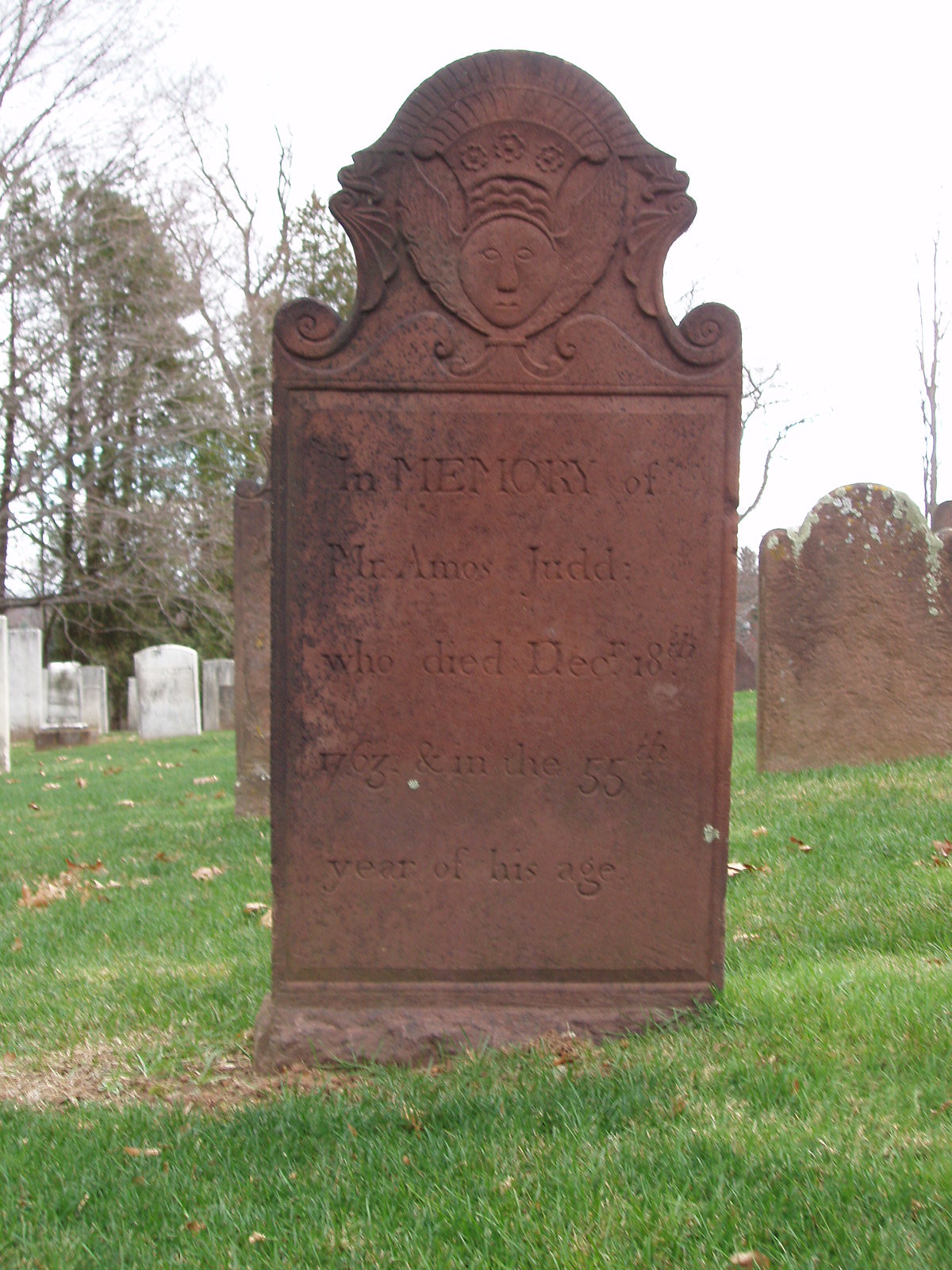The image showcases a weathered and rusted grave marker set in an inclined grassy field scattered with dead leaves, indicating the autumn season. The bronze-colored tombstone, adorned with a carved head featuring wings and scroll decorations at the top, is dedicated to Mr. Amos Judd, who died on December 18, 1703, in the 55th year of his age. The weathering has rendered parts of the inscription difficult to read. The scene includes additional tombstones, both red and grey, some covered with moss or plants. Behind these grave markers, trees, some lush and some bare, stand under an overcast white sky, emphasizing the somber atmosphere of the graveyard during the daytime.